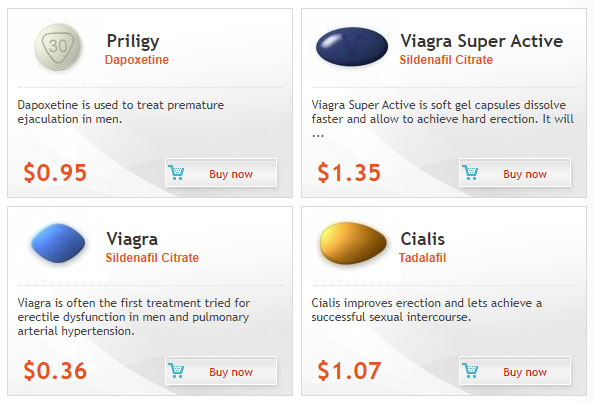The image showcases a selection of pills available for purchase, arranged in a grid of four panels, with two panels on top and two on the bottom. Notably, the image lacks any branding or website header. 

The first panel features Priligy, which is also known as Dapoxetine. This medication is used to treat premature ejaculation in men and is priced at 95 cents per pill. The pill is round and embossed with the number "30".

The second panel highlights Viagra Superactive, a blue, lozenge-shaped pill. This brand-name medication, containing Sildenafil Citrate, is priced at $1.35 per pill.

The third panel shows another variant of Viagra, also a lozenge-shaped, light blue pill, but this one is priced at 36 cents per pill, indicating it is not the Superactive version.

The fourth panel presents Cialis, a golden, teardrop-shaped pill. Its generic name is Tadalafil, and it is priced at $1.07 per pill.